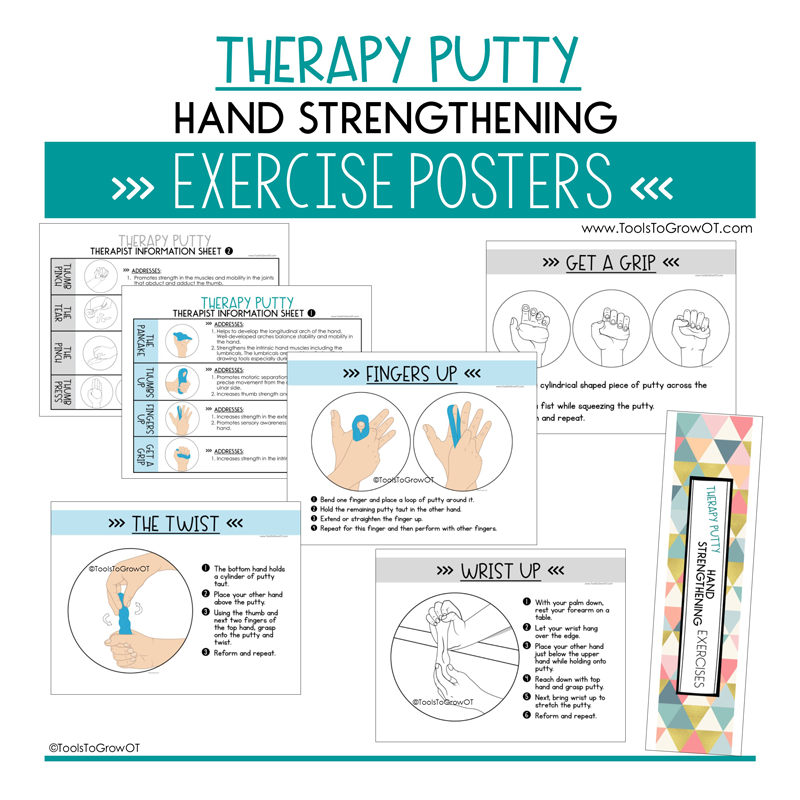The image is a detailed infographic poster with a white background and organized sections. At the top, "Therapy Putty" is prominently displayed in greenish-blue, underlined in the same color. Directly below, in black capital letters, it reads "Hand Strengthening." A teal-colored rectangle spans across the middle with "Exercise Posters" written in white, flanked by arrows pointing towards the text from both sides.

Beneath this header, the poster features various rectangular exercise diagrams. On the left side, three diagrams are arranged diagonally. The middle one, labeled "Fingers Up," displays two images of hands with associated exercises and descriptions in black text. Above it to the left, a card titled "Get a Grip" shows three stages of a hand grip with corresponding images and instructions. Below on the left, another card is labeled "The Twist," featuring two hands holding and twisting an object, depicted within a circular graphic and explanatory text to the right.

On the bottom right, a diagram labeled "Wrist Up" includes an image within a circle on the left side and descriptive text on the right. Adjacent to the wrist exercise is a tall rectangle colored with triangles, featuring a white outlined box containing indistinct text. 

At the base of the infographic, the company's name or copyright information is presented within a greenish-blue line at the bottom.